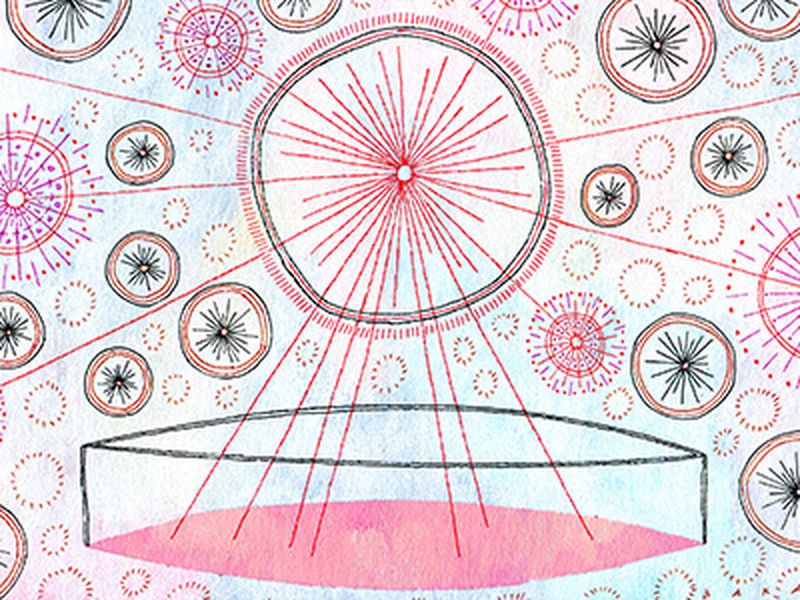The image displays a collection of predominantly circular shapes, set against an almost whitish blue background, suggesting it is some form of drawing. The focal point is a large circular object near the center but slightly towards the top. This central shape has a black center surrounded by fringe resembling pinkish-red hues, from which spritzes of red lines radiate outward, reminiscent of a firework. These lines extend throughout the image, converging towards the base where they enter a semi-cylindrical structure filled with red liquid and capped with white. Surrounding the main circle, there are multiple smaller circular objects, some with star-like or swirly structures, often outlined in black or green. The colors in the image consist of red, purple, blue, and black, with many of the smaller shapes being undefined and broken around their edges.